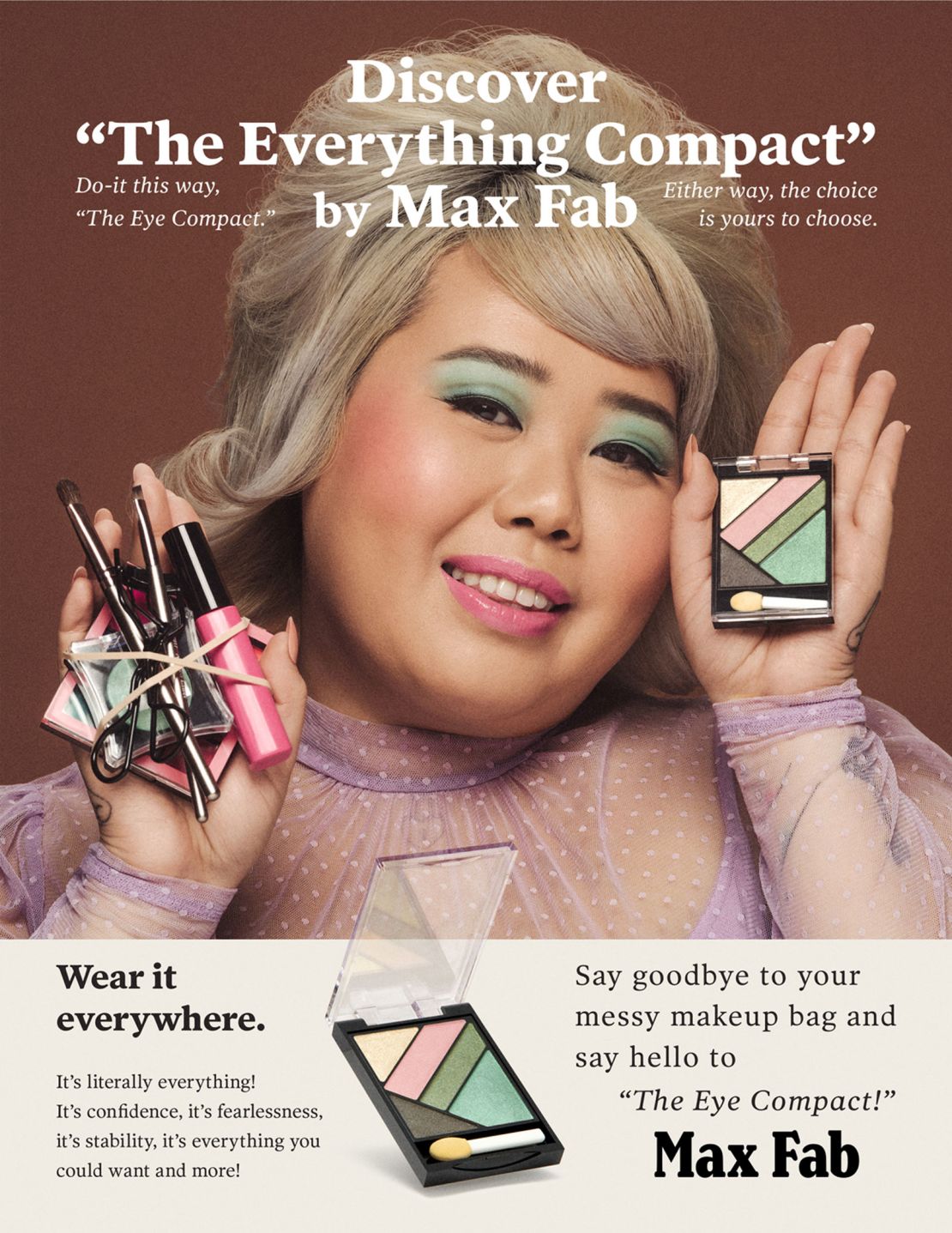In this vibrant makeup advertisement poster for Max Fab's "Everything Compact," a smiling woman with slightly darker skin and a 1960s-inspired short blonde hairstyle appears at the forefront. Her face is adorned with pink lipstick, green eyeshadow, brown eyebrows, and a subtle blush on her cheeks. She wears a lavender organza dress that enhances the retro aesthetic. In her right hand, she clutches a collection of assorted, rubber-banded makeup containers she seemingly no longer needs. In her left hand, she proudly displays the featured Max Fab Everything Compact, an all-in-one makeup kit containing colors such as cream, pink, green, blue, and gray, along with a small brush. 

The ad features white text across the top that reads, "Discover the Everything Compact by Max Fab," with the phrase "Everything Compact" in quotes. The bottom portion of the poster showcases the open compact, emphasizing the convenience and variety of the kit. Below this image, it declares in black text, "Wear it everywhere. It's literally everything." Adjacent to it, in a smaller font, it reads, "Say goodbye to your messy makeup bag and say hello to the Eye Compact." The bottom right corner of the ad is marked with the brand name, "Max Fab," in bold black text.